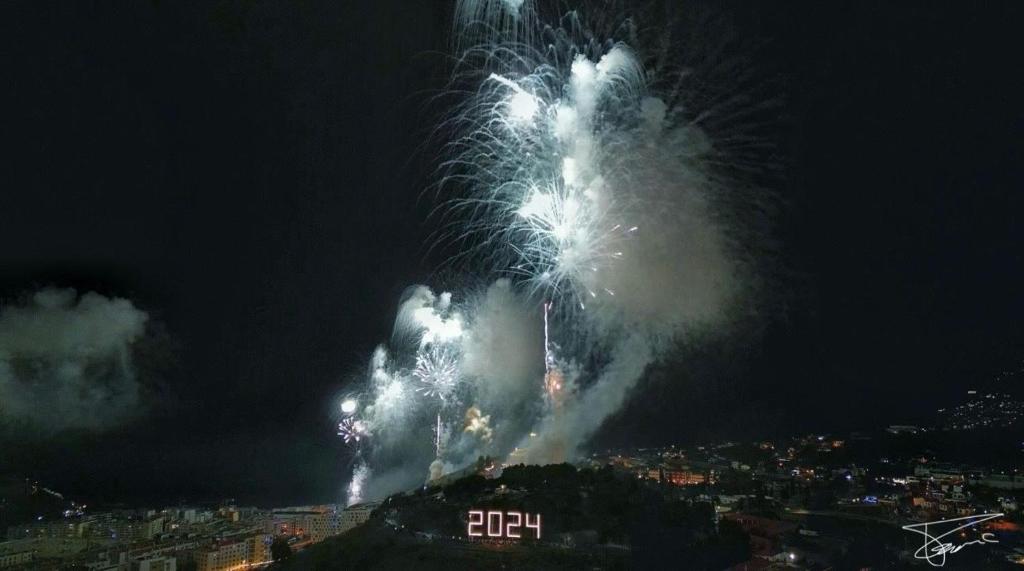The image captures a vibrant nighttime fireworks display exploding above a hill, with the sky around it filled with bright, colorful flares and billowing clouds of smoke. In neon red, "2024" is prominently displayed near the base of the hill, marking the year of the celebration. The scene is viewed from a considerable distance, suggesting the photographer was positioned in a tall building far away from the action. The dark hill, dotted with trees, serves as the launch point for the fireworks, while below it, the silhouettes of some beige, standard block apartment buildings and additional city structures delineate the backdrop. Off to the left, more detailed cityscape elements with numerous illuminated lights can be discerned, adding context to the festive scene. A barely readable signature is situated at the bottom right corner of the photograph, underscoring its artistic authenticity.